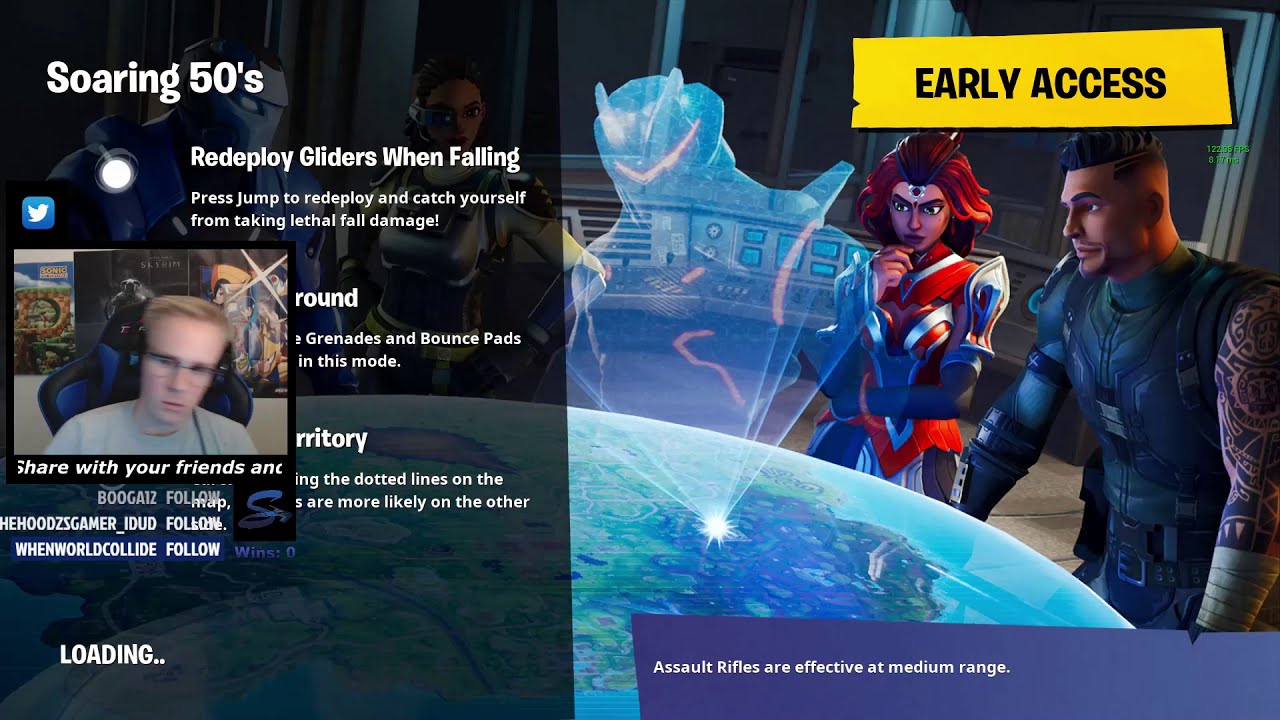This is a screenshot of a YouTube gamer playing a video game on their computer or console. The game is in "Early Access," as indicated at the upper right corner. The scene features an animated background where a man and a woman stand by a luminescent, blue globe. The globe has a bright light projecting an image resembling a genie or robot. The man, who has a black armor-like outfit and a tattoo on his left arm, stands beside the woman wearing a red and white striped bodysuit. In the upper left corner, the text reads "Soaring 50s," followed by instructions about redeploying gliders while falling to avoid lethal fall damage. There is additional text about game mechanics like grenades and bounce pads. The lower right corner message advises that "Assault rifles are effective at medium range," while "Loading" is displayed in the lower-left corner. A small square photo of the YouTuber, wearing a gray shirt, with blonde hair and eyeglasses, is positioned at the middle left of the screen. Above him is a Twitter icon.